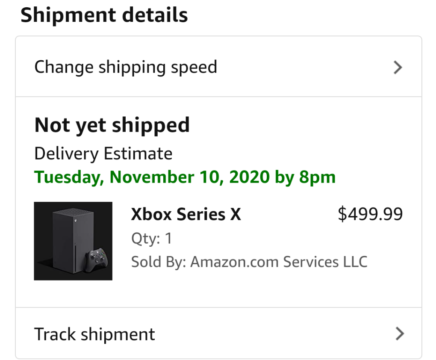**Shipping Details: Xbox Series X Order**

At the top left of the panel, bold text reads "Shipping Details." Directly below this section, there is an option labeled "Change shipping speed" with a rightward arrow icon. Here you can adjust your shipping preferences.

The next section states "Not shipped yet" and "Not yet shipped" in bold black letters. Beneath this, in green text, the delivery estimate is provided as Tuesday, November 10th, 2020, by 8 p.m.

The order item is detailed as an image of a gray vertical tower with a controller beside it, labeled "Xbox Series X." The listed price is $499.99, with a quantity of one unit, sold by Amazon.com Services LLC. A thin gray line separates this information from the other sections.

An option to "Track shipment" is provided below a similar rightward arrow icon. This information is set against a white background, and everything under the "Shipping Details" header appears on a floating panel outlined with a thin line, with separators above and below pertinent sections.

Though this document is not an order confirmation, it details the current shipping status and provides options to adjust or track the order.